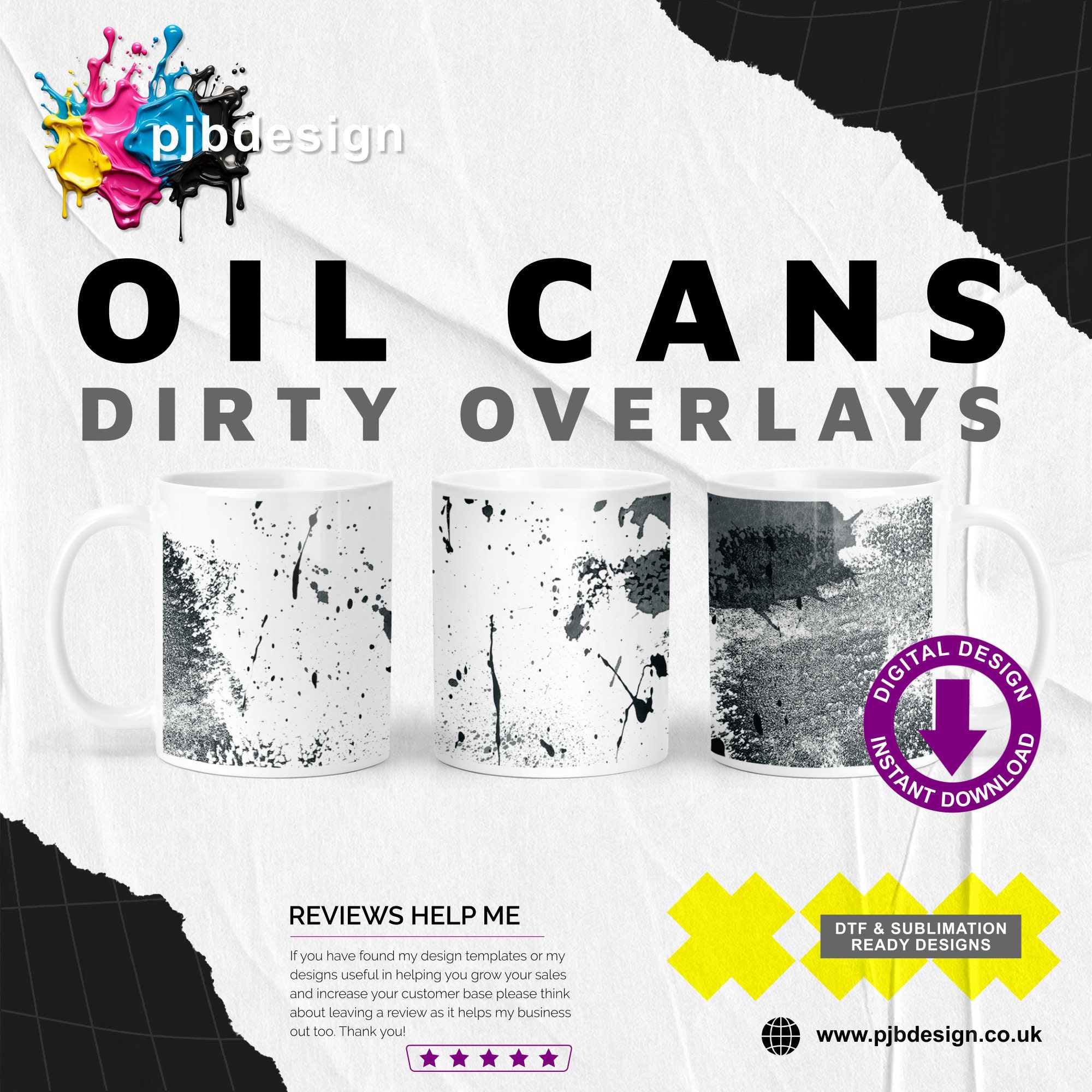The black and white advertisement image for PJB Design features a stark, mostly white backdrop with contrasting black sections in the upper right and lower left corners. Positioned prominently in the upper left corner is the artist's vibrant logo, composed of splatters of yellow, teal, pink, blue, and black paint, with "PJB Design" written in white. Central to the image in bold black uppercase letters is the title "OIL CANS," followed below by "DIRTY OVERLAYS" in dark gray uppercase letters. 

The focal point showcases three white coffee mugs decorated with the 'Oil Cans Dirty Overlay' design, which includes abstract, splatter-painted patterns in various shades of gray and black. Notably, the third mug on the right features the most detailed design, giving the impression of a tangible image rather than all-over splatterings. Adjacent to this mug is a purple circle containing "Digital Design Instant Download" in white text, with a downward-pointing arrow directing towards three yellow Xs that state, "DTF Sublimation Ready Designs" within a gray box.

At the bottom, slightly left of center, a black text prompts viewers: "REVIEWS HELP ME." Below this, it reads, "If you have found my design templates or designs useful in helping you grow your sales and increase your customer base, please think about leaving a review as it helps my business out too. Thank you." To the right of this message is a globe icon accompanying the web address www.pjbdesign.co.uk. Additionally, a set of purple stars is enclosed in a box, inviting viewers to rate and review the product.